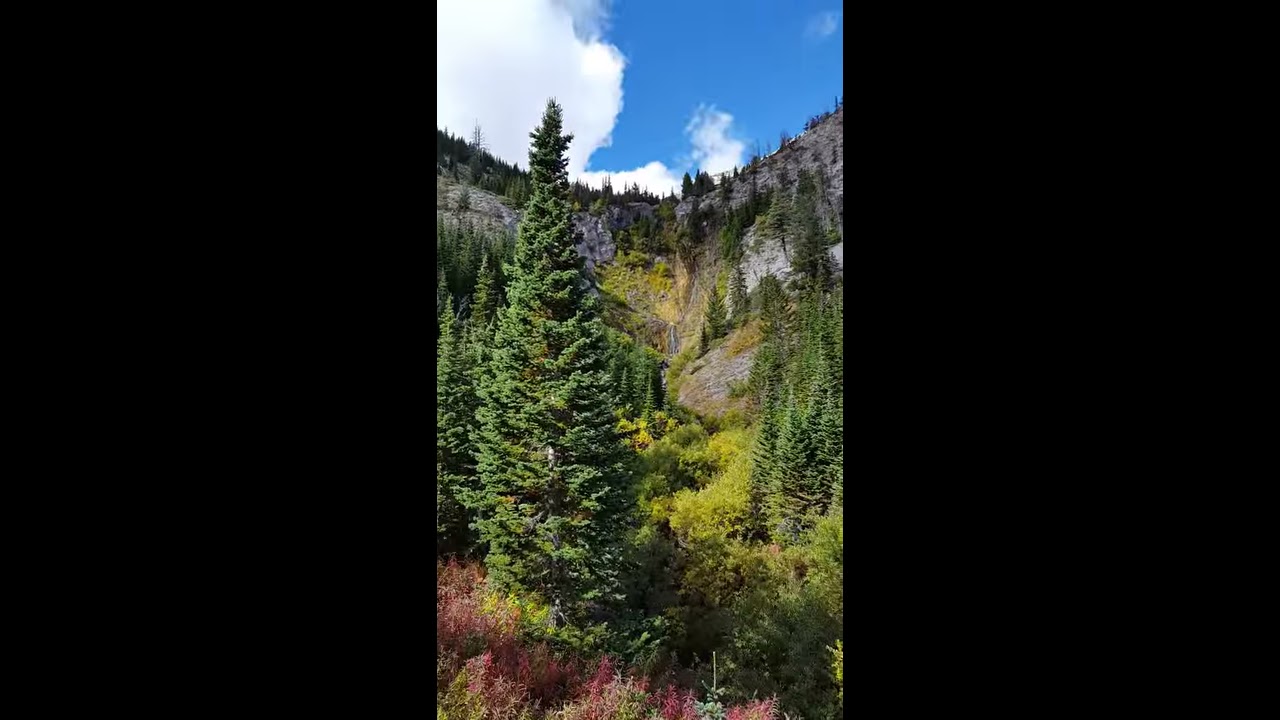The image captures an invigorating mountain landscape viewed from a valley. At the forefront, there is a patch of wheat in shades of dull red and brown, interspersed with patches of wildflowers in red and pink. A steep path winds up the hill, adorned with a mixture of dark and light green bushes. Dominating the foreground is a strikingly large pine tree, leading the eye up the rocky hillside dotted with an array of robust pine trees. Gray and white rocks feature prominently at the hill's peak. Above this vibrant scene, a brilliant blue sky stretches, punctuated by fluffy white clouds, casting a serene backdrop over the rich, dynamic natural environment. The edges of the image have a subtle black border, framing the vivid outdoor scene within.